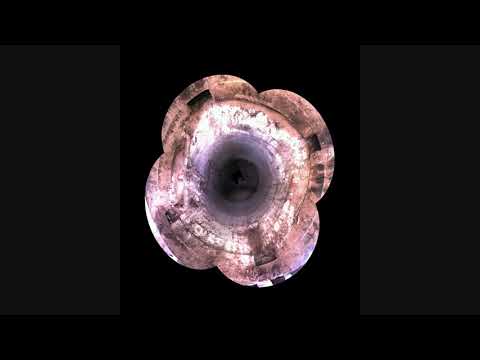The image depicts an ancient, rusted bowl viewed from a top-down angle against a black background, occupying roughly 75% of the frame. The bowl has four small curved indentations around its rim, creating overlapping circular shapes that present a visual effect reminiscent of an eye or planetary surface. The rim showcases lighter-colored rings fading into darker, grayish tones as they progress inward. The base of the bowl is significantly darker, almost black, accentuating its shallow depth. Indistinguishable letters are scattered across the bowl's surface, heavily marked by pronounced rust, particularly around the indentations. This intricate blend of white, brown, and darker hues against the stark background highlights the bowl's aged and mysterious appearance.